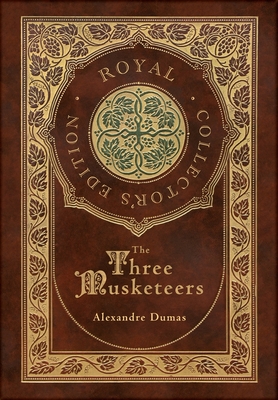The cover of this Royal Collector's Edition of "The Three Musketeers" by Alexandre Dumas features a rich brown background adorned with intricate gold decorative elements. A prominent rectangular inset, bordered by a wavy pattern of leaves, encloses the title and author's name. 

At the top of the inset, a circle encases the words "Royal Collector's Edition," surrounded by ornate golden leaves and bunches of grapes, with a greenish hue highlighting this area. Below this circle, the title "The Three Musketeers" and the author's name "Alexandre Dumas" are prominently displayed. 

The design is characterized by its elaborate embellishments, including gold entwinement and a green Maltese-like cross that adds to the book's luxurious and collectible appearance.